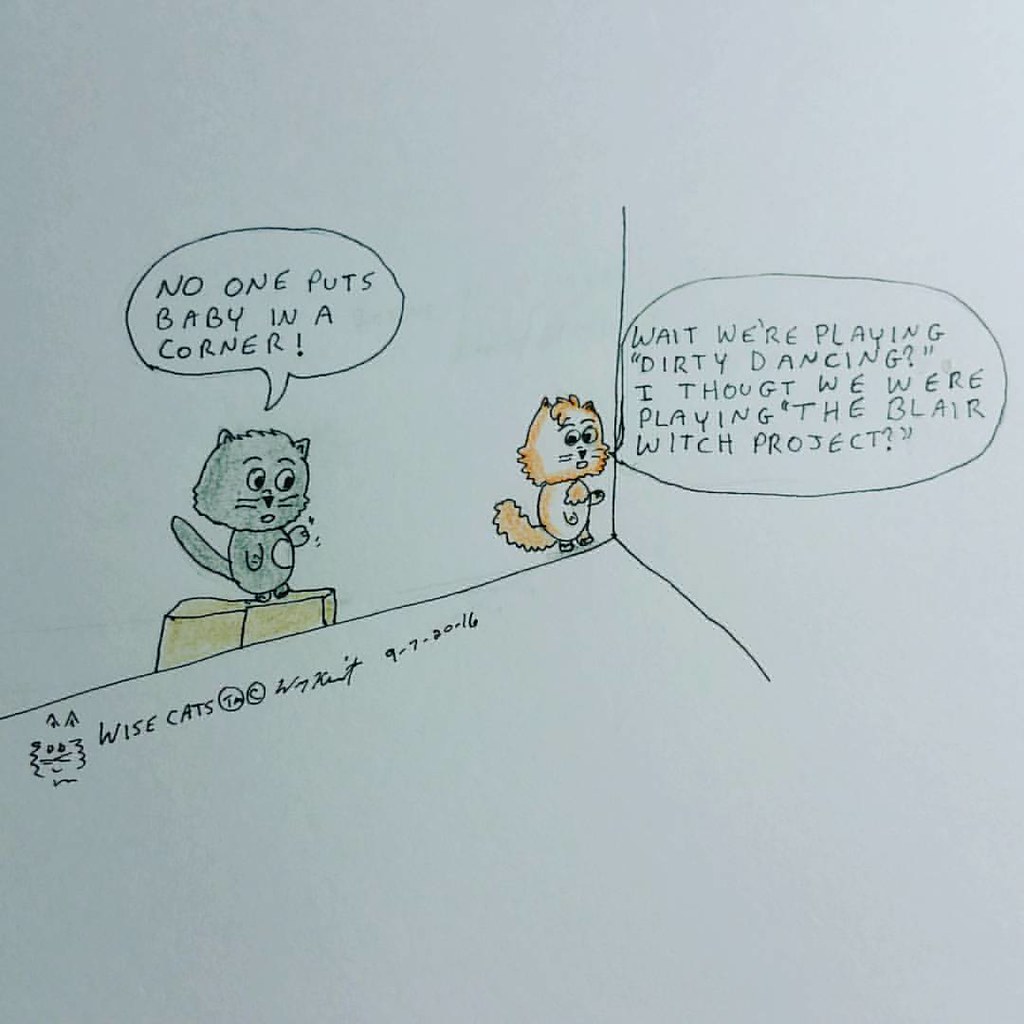This hand-drawn cartoon features two cats in the corner of a room, depicted in a sketch with light color on what appears to be printer paper. The background is white, drawn with a fine point pen or marker, and shows two deformed walls intersecting at right angles. On the left wall stands a grey cat atop two yellow blocks with a speech bubble that reads, "No one puts Baby in a corner!" Opposite him, at the intersection of the walls, an orange-brown cat responds with, "Wait, we're playing Dirty Dancing? I thought we were playing The Blair Witch Project." Below the grey cat, there is a small hand-drawn cat face icon accompanied by the text "Wisecats," a trademark symbol, and the date September 7, 2016, including what seems to be the artist's signature.